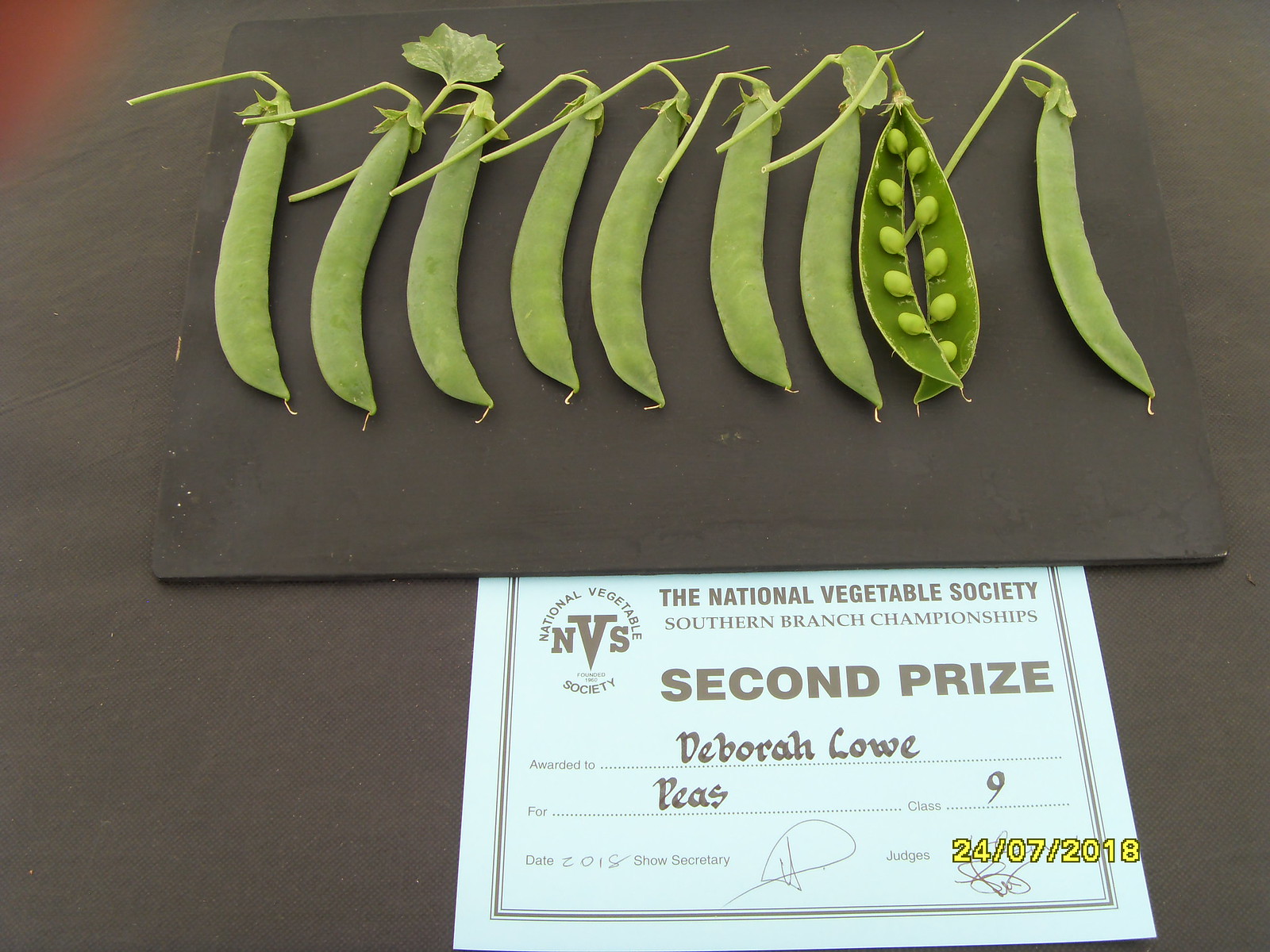In this photo, a collection of meticulously arranged green vegetables, specifically peas, lie on a brown mat placed over a brown tablecloth. There are ten pea pods in total: nine unopened ones neatly lined up and one split in half to reveal ten peas inside, showcasing their perfect form. Just below this arrangement, there's a light blue card with the text "Second Prize" and recognizing Deborah Lowe for her entry in the National Vegetable Society Southern Branch Championships, Class 9 category for peas. The card includes signatures from the judges and features the logo of the National Vegetable Society Southern Branch. The date "24-07-2018" is prominently displayed in yellow text with a black outline, indicating the event took place in the summer of 2018.